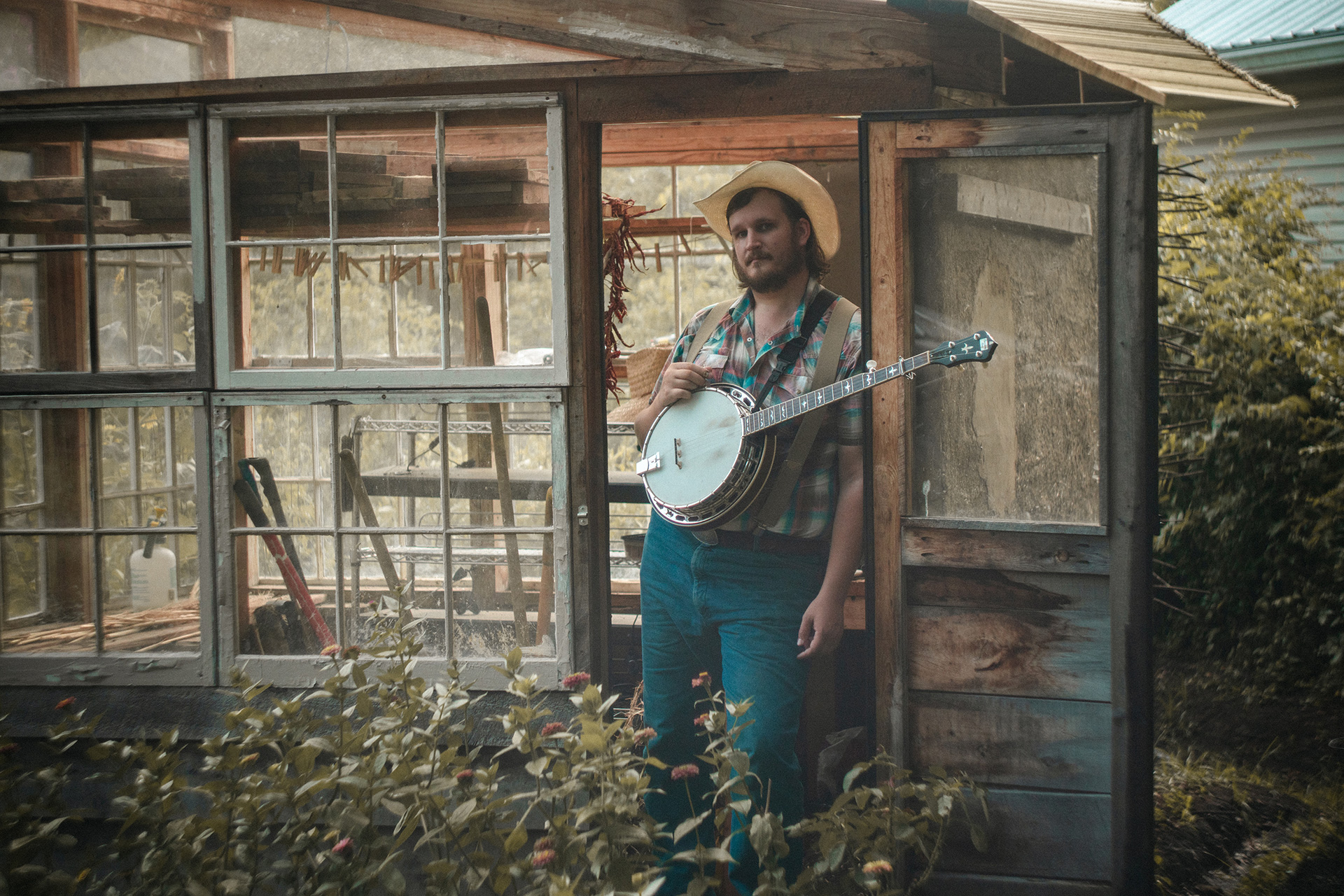In this detailed photograph, a man stands prominently, visible from the knees upwards. He is dressed in blue denim jeans secured with a brown leather belt that features an oval-shaped silver buckle. His pants are further held up by tan suspenders adorned with silver buckles fastened to the top of his pants. He sports a white, blue, and pink plaid short-sleeved shirt with a button-up front, with the top two buttons undone, giving a relaxed appearance. Atop his head is a white straw cowboy hat, and around his neck is a black nylon strap attached to a round white banjo with a black neck.

He is positioned in what appears to be a rustic greenhouse, evidenced by the structure's original green paint now faded and revealing the wood beneath. The greenhouse is characterized by its numerous glass windows, one of which reveals glimpses of green plants outside. The background also hints at features of a wooden cabin, specifically a nearby door with a glass window that stands open, contributing to the airy and worn yet charming ambiance of the setting.